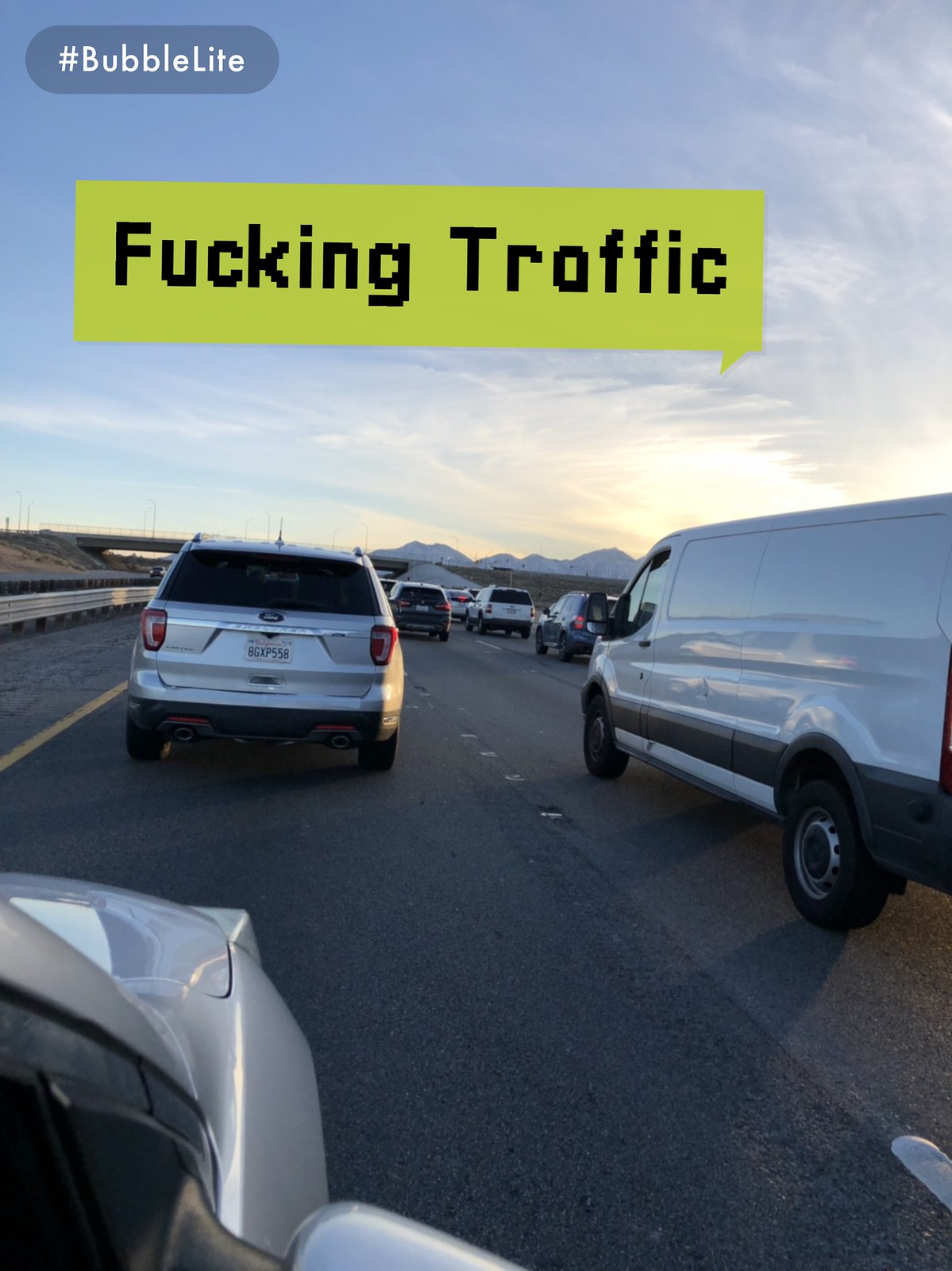The image depicts a scene of bumper-to-bumper traffic taken from the perspective of a passenger inside a car. In the foreground, a Ford vehicle with the license plate AGXP558 is prominently visible, among several other cars ahead, including a white minivan, a blue car, and a BMW. The sky is a clear blue with a few scattered clouds, indicating it's a sunny morning, possibly around sunrise. 

A notable feature in the picture is a green pixelated speech bubble with black text that graphically expresses the frustration of the situation with the words "fucking traffic." In the top left corner, there's a yellow hashtag bubble followed by the word "bubblelight," suggesting the photo may have been posted on social media or taken with an app that adds such effects. The scenery suggests an arid climate, likely in the southwest United States, and shows multiple lanes of stationary vehicles heading towards an underpass with a road overhead.